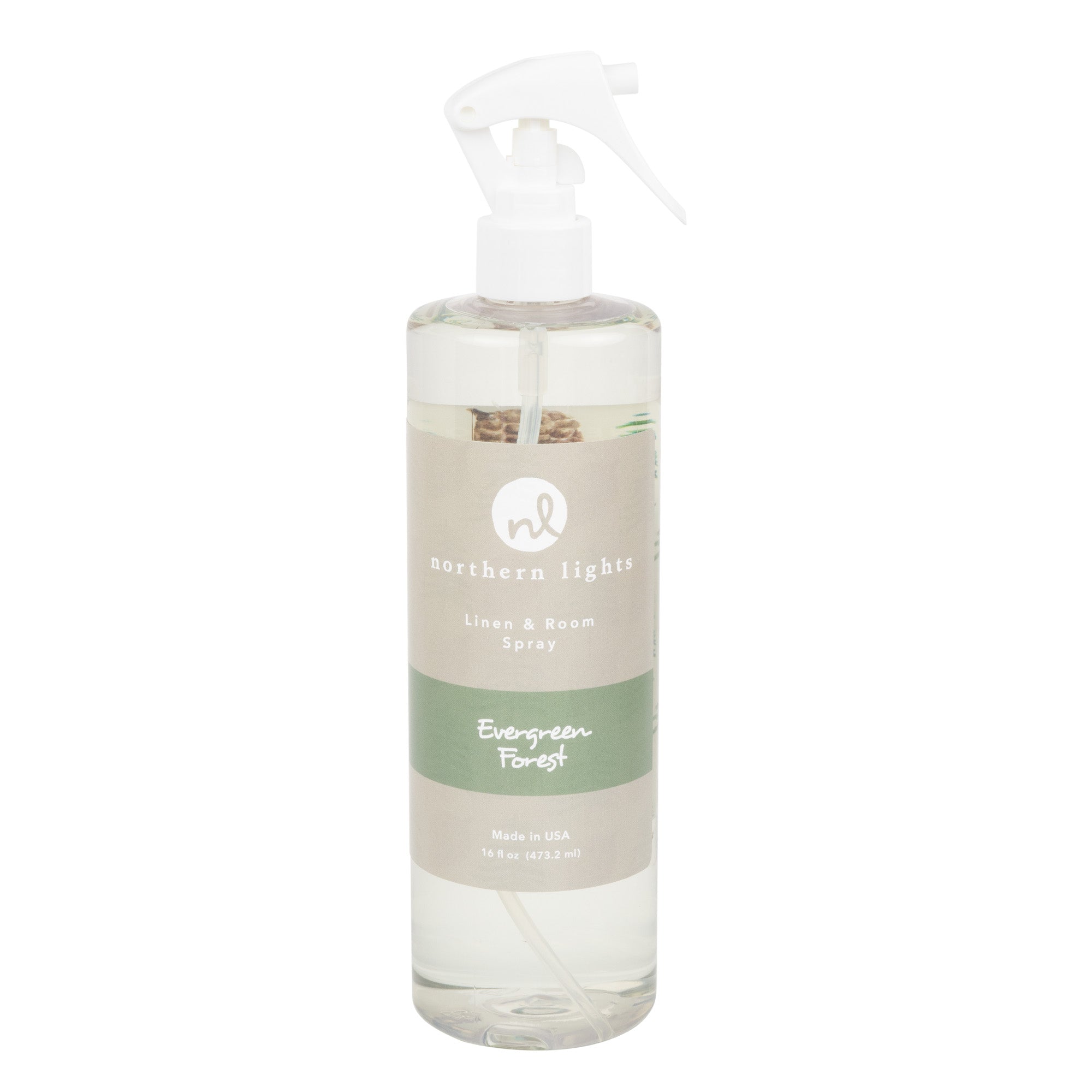The image showcases a linen and room spray bottle set against an entirely white background. The bottle is tall and skinny, made of clear plastic, revealing the transparent liquid inside. The white spray nozzle at the top points to the right. The bottle features a beige-gray label adorned with several details. At the top of the label, there's a circular logo with the cursive letters "NL." Below this, the brand name "Northern Lights" is written, followed by the description "Linen and Room Spray." Towards the bottom of the label, a light forest green band displays the scent name "Evergreen Forest" in white cursive font. Beneath this green strip, it states, "Made in USA, 16 fluid ounces (473.2 milliliters)."